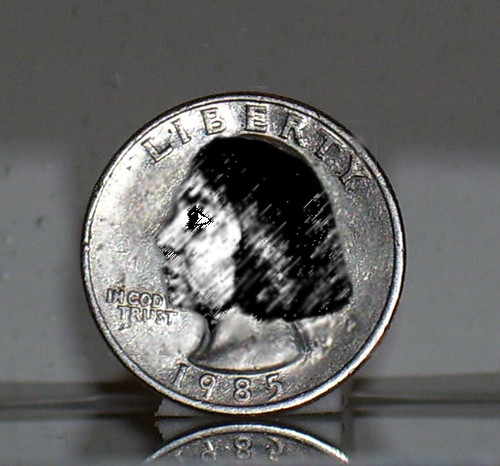This image features an altered 1985 quarter shown in an extreme close-up. The quarter, which typically depicts George Washington, has been edited to display a woman with dark black hair, possibly of Middle Eastern or African-American descent. Her hair is long, just above her shoulders, and feathers out in the back. Her eyes are prominently black and wide open. The coin retains its original raised silver letters, reading "LIBERTY" at the top and "1985" at the bottom. Additionally, the phrase "In God We Trust" is partially obscured by the woman's chin, appearing around the eight o'clock position. The coin is positioned upright on a reflective glass or mirrored surface, creating a clear reflection of its bottom half. The background behind the coin is a plain white wall, which contrasts with the coin's detailed, professionally altered visage.